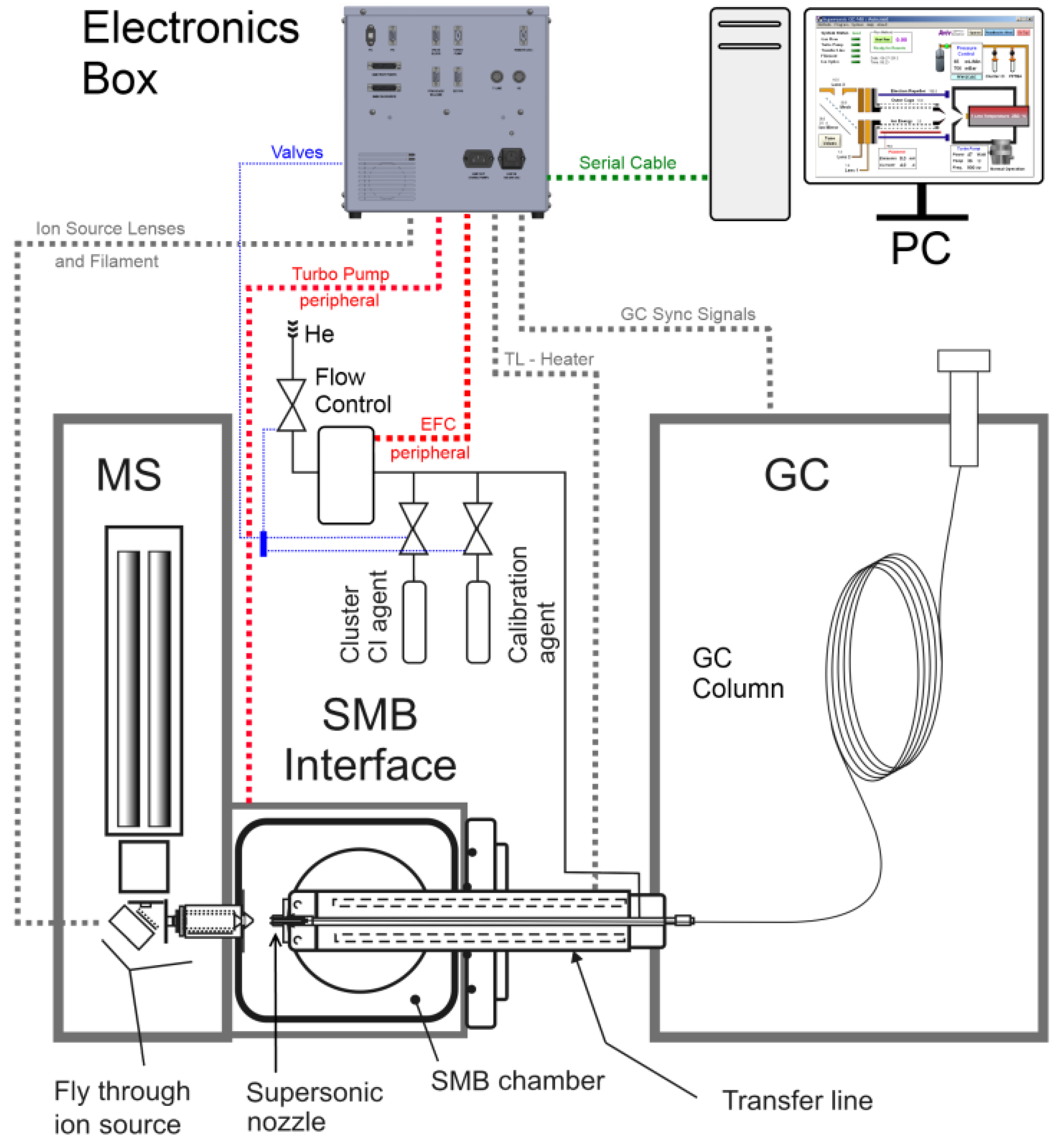This image illustrates a detailed electronic diagram on a white background. In the upper left corner, a black-labeled "Electronics Box" connects via a green-dotted line, labeled "Serial Cable," to a nearby desktop computer (CPU) and a PC monitor displaying a colored schematic. Blue-dotted lines extend from the "Electronics Box" to valves and a "Cluster CI Agent" and "Calibration Agent." A black-dotted line links the "Electronics Box" to "Ion Source Lens and Filament," leading to a gray-bordered rectangle marked with "MS" and the words "Fly Through Ion Source."

At the center of the diagram, a red-dotted line labeled "Turbo Pump Peripheral" branches out alongside another bold red line identified as "EFC Peripheral." A separate gray-dotted line from the "Electronics Box" to the lower section indicates "GC Sync Signals," with another gray line marked "TL Heater."

On the lower right, a prominent gray-bordered rectangle titled "GC" houses a "GC Column" and is connected through multiple lines, showing integrations across the system. Below this area, the diagram illustrates components such as a "Supersonic Nozzle" and an "SMB Chamber," encapsulated within an "SMB Interface."

Overall, this schematic maps out the intricate connections and functionalities within the electronic system, highlighting various control and transfer lines, peripheral devices, and essential components.